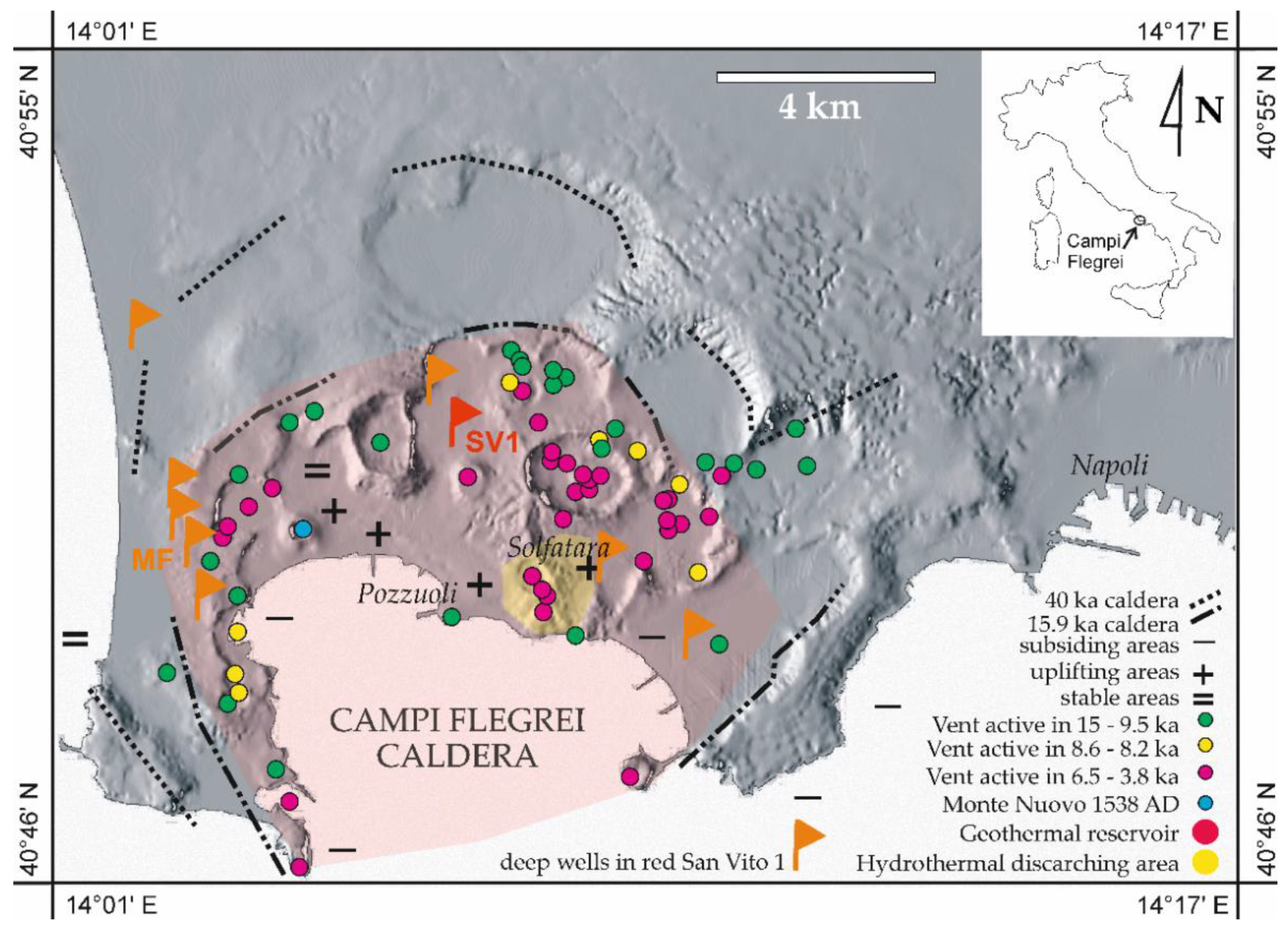The image features a detailed topographic map primarily shaded in gray, depicting the Campi Flegrei Caldera located in the lower left-hand region of Italy. The map includes various marked features in colors such as pink, green, yellow, blue, and red. A smaller, outlined map of Italy is positioned in the upper right corner for geographical context, highlighting the location of the caldera.

This map comes with a comprehensive key on the right side, explaining the significance of the colored markings. Yellow, pink, and green dots indicate different geothermal and geological features like subsiding areas, uplifting areas, stable areas, and vents active during specific prehistoric periods. Notably, it references features such as the 40KA and 15.9KA calderas, a geothermal reservoir, and hydrothermal discarding areas.

Some key points are:
- The section circled in pink marks the Campi Flegrei Caldera.
- Green and pink dots are scattered around the map indicating various geological features.
- Different periods of volcanic activity are noted, including vents active between 15 to 9.5KA, 8.6 to 8.2KA, and 6.5 to 3.8KA.
- The map provides information in Italian, further affirming its international origin.

Overall, the map serves as an informative geospatial representation of the dynamic geological features and historical volcanic activity of the Campi Flegrei Caldera in Italy.